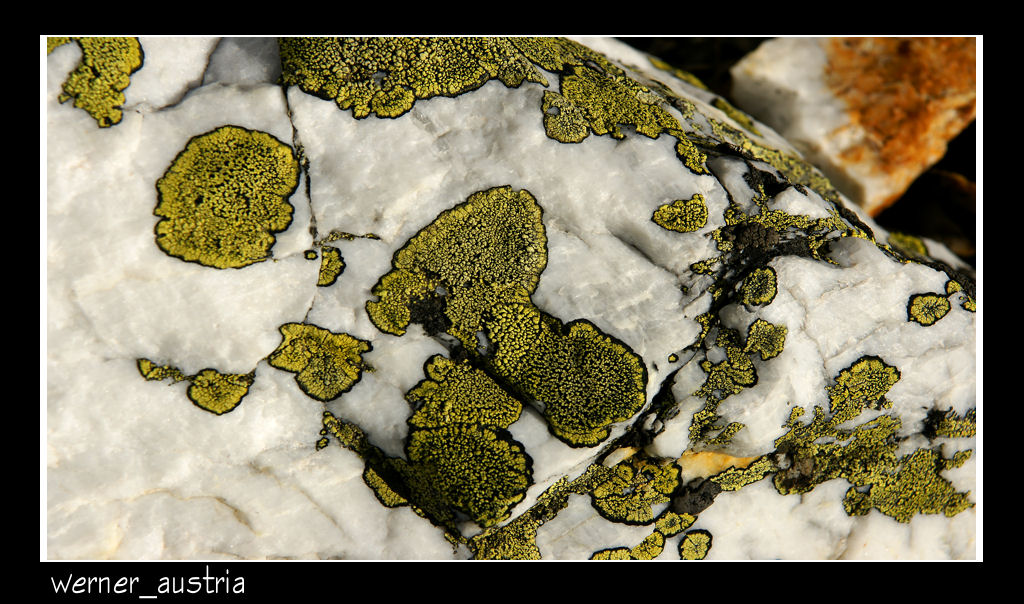This photograph, bordered in black with the text "Werner_Austria" in the lower left corner, captures a detailed close-up of a white, textured stone or rock. The stone appears somewhat rounded and rugged, evocative of granite, and is predominantly white with multiple green patches suggestive of mold or algae growth. These green patches vary in size and texture, exhibiting splotches that range from tiny dots to larger, smeared areas, with some having a slimy appearance in green and yellowish hues. In the upper right corner of the image, there appears to be another object that looks like a piece of bread or stone with orange and white coloration, adding to the complex visual texture of the scene. The photograph's detailed textures and variable organic growth give it a somewhat unsettling yet intriguing character.